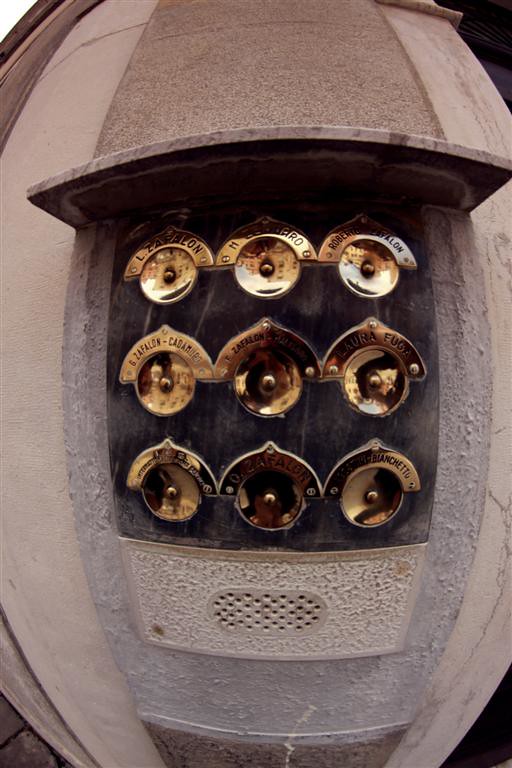The photograph showcases the side of a beige stone building, featuring a centered small overhang canopy. The canopy shelters nine golden-colored metal bells arranged in a three-by-three grid. These elements, which appear to function as doorbells or buzzers, each have a half-horseshoe shaped bar above them with inscriptions or names, though the text is not discernible. At the center of each bell is a small pin. Mounted below this grid is a rectangular gray structure resembling a speaker, with multiple holes for sound transmission. The overall appearance suggests these are used to signal apartments within the building.